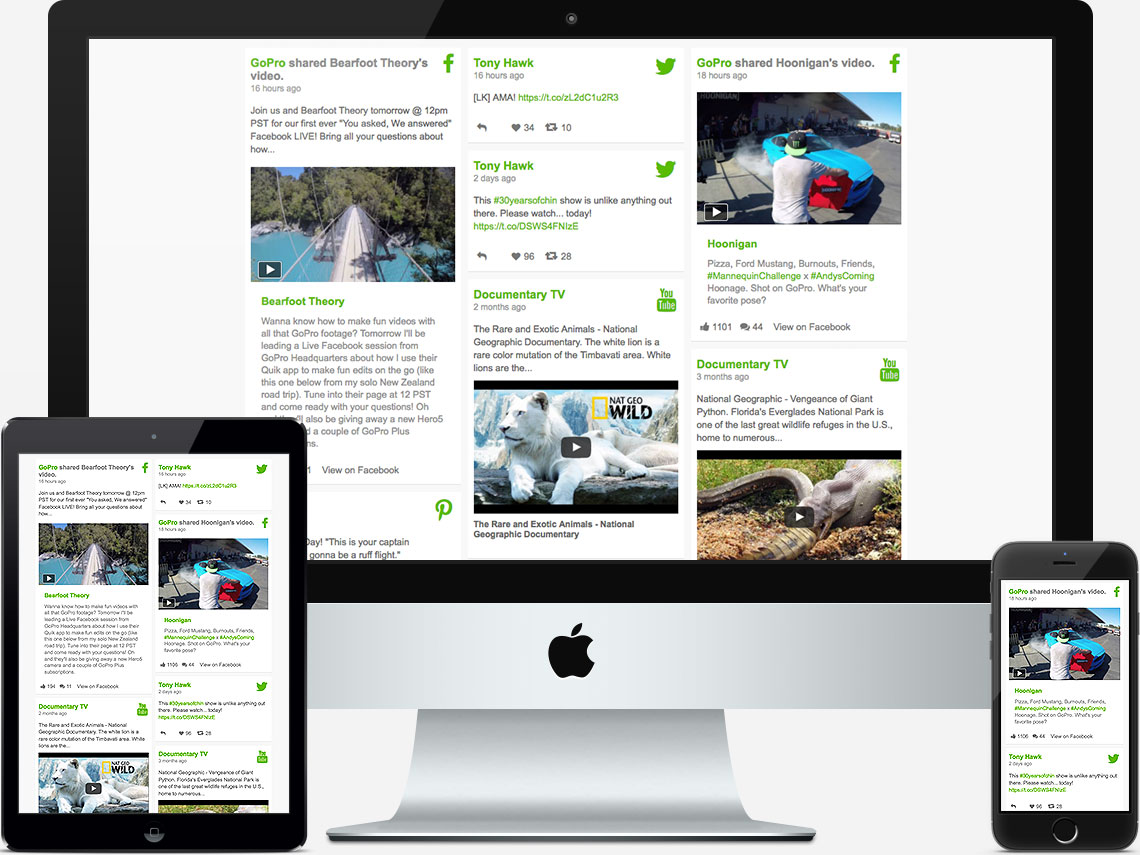This image showcases a neat display of multiple Apple products arranged in a workspace setting. In the background, a sleek silver computer monitor with an integrated stand dominates the scene. The monitor, which seems to be an iMac due to its unified design, features the distinctive black Apple logo centered at the bottom of its bezel. In front of the monitor, oriented slightly to the left, is an iPad positioned upright, partially obscuring a portion of the monitor. Completing the trio is an iPhone placed vertically to the right of the iPad. All three devices are powered on and displaying the same webpage, which appears to be filled with text and images, though the content is not entirely clear. The setup illustrates a cohesive ecosystem of Apple products working in harmony within a modern and organized digital environment.